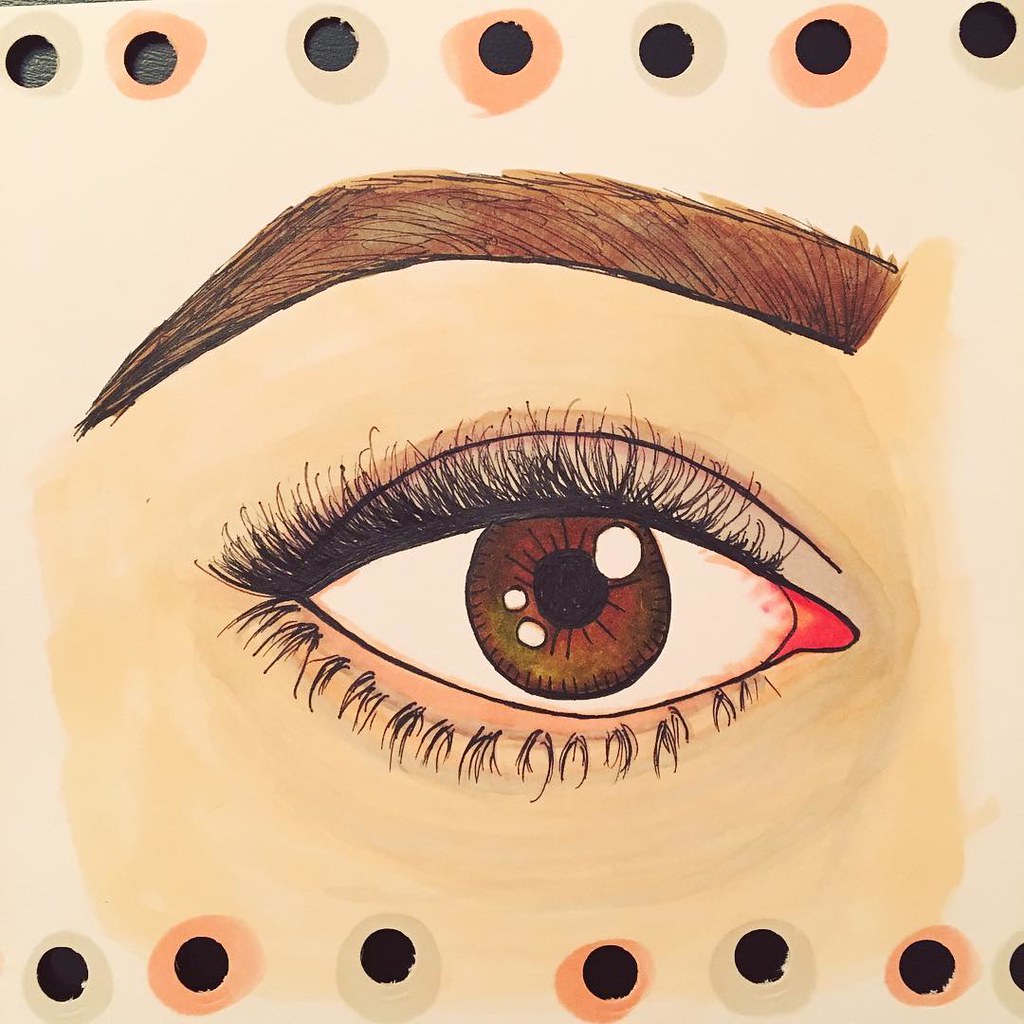The image features a finely rendered watercolor and marker illustration focusing on a person's right eye. The skin tone is a light tan, providing a soft backdrop to the central eye, which appears in rich shades of brown with hints of green. Surrounding the eye, the lashes are meticulously detailed in black.

Above and below the eye, there are rows of seven circular holes. These punched-out details reveal a horizontally jagged, almost leather-like black laminate surface beneath the drawing paper, suggesting the drawing is placed on a desk with a textured, imitation leather finish. The holes' edges are decorated in alternating light gray and pink hues, starting with gray.

The upper left corner of the image reveals part of this black laminate surface, enhancing the textured aesthetic. The eye's deep expression is complemented by the artist's delicate strokes, making the fine details like the eyelashes and the slight color gradient in the iris stand out.